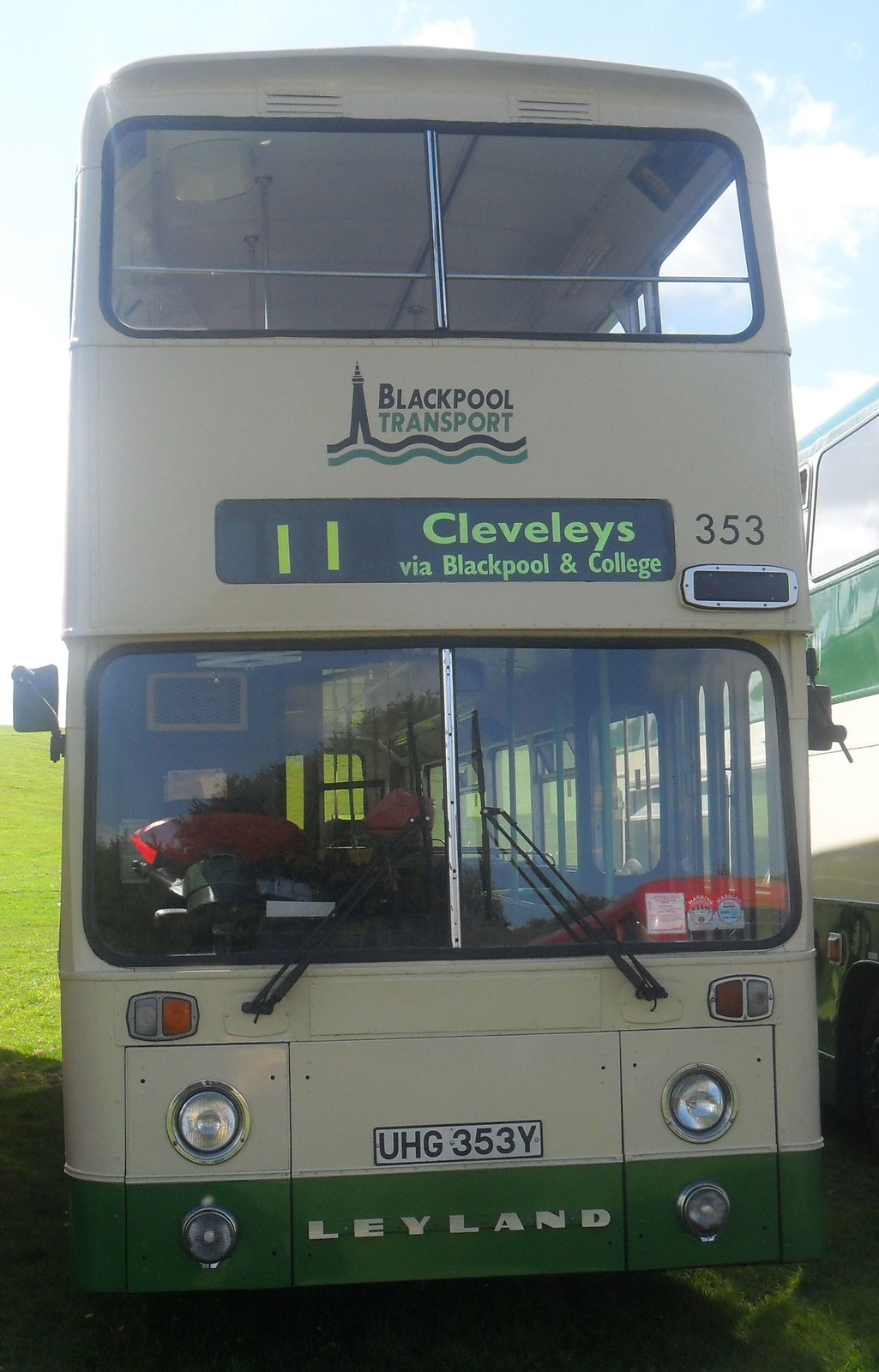The image features the front view of a vintage, cream-colored double-decker bus with a distinctive green line running along the bottom. The bus, part of the Blackpool Transport fleet, prominently displays "Blackpool Transport" in black and green on a panel between the two front windows. Above the front window, there is a route indicator stating "11 Cleveleys via Blackpool and College" along with the number "353" painted nearby. The front of the bus also showcases its number plate, "UHG 353Y", set against a white background with black letters. The bus boasts circular headlights with two larger ones positioned vertically above the smaller ones on each side. 

Additionally, the bus carries the brand name "Leyland" in cream on a green banner at the bottom, accompanied by indicator lights above the side lights. The image shows the driver's seat on the left and a glimpse of the bus's right and left side interior through the windows, where a red object, possibly a steering wheel cover, and something pink can be seen. The background of the image features a white sky and green grass partly shadowed by the bus, with another bus partially visible on the right side of the frame.